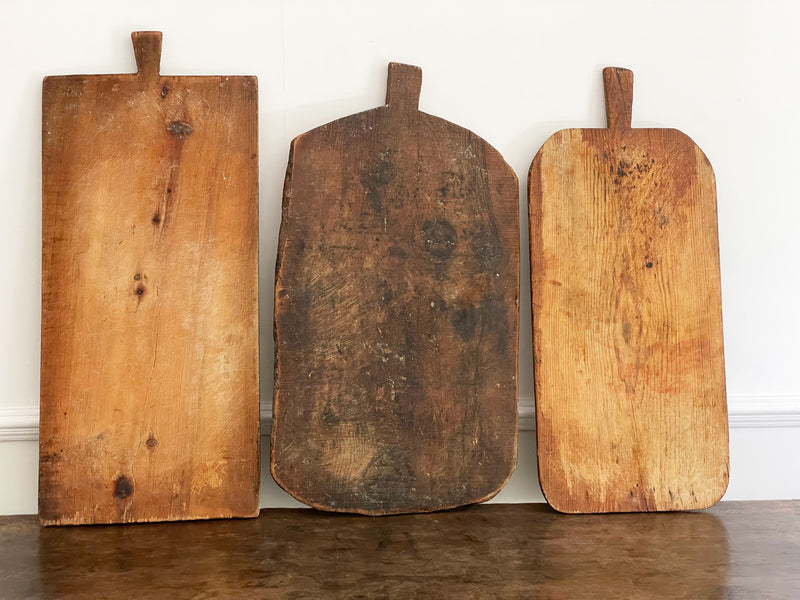This photograph showcases three distinct wooden cutting boards of varying woods and sizes, leaning against a pristine white painted wall with a white base frame. The boards rest on a dark brown polished wood floor with darker brown spots. The leftmost cutting board is rectangular and crafted from a medium reddish-brown wood, prominently marked with black knots and various scratches, giving it a worn appearance. It features a small, unique triangular notch or handle at the top. The central cutting board is darker and more roughly hewn with oval, rounded edges and a small handle, suggesting a robust, handmade quality. The rightmost board is the narrowest, a lighter brown with a rectangular shape and rounded edges. Its handle is slightly longer compared to the others. Each cutting board tells a story of use and craftsmanship, adding rustic charm to the scene.